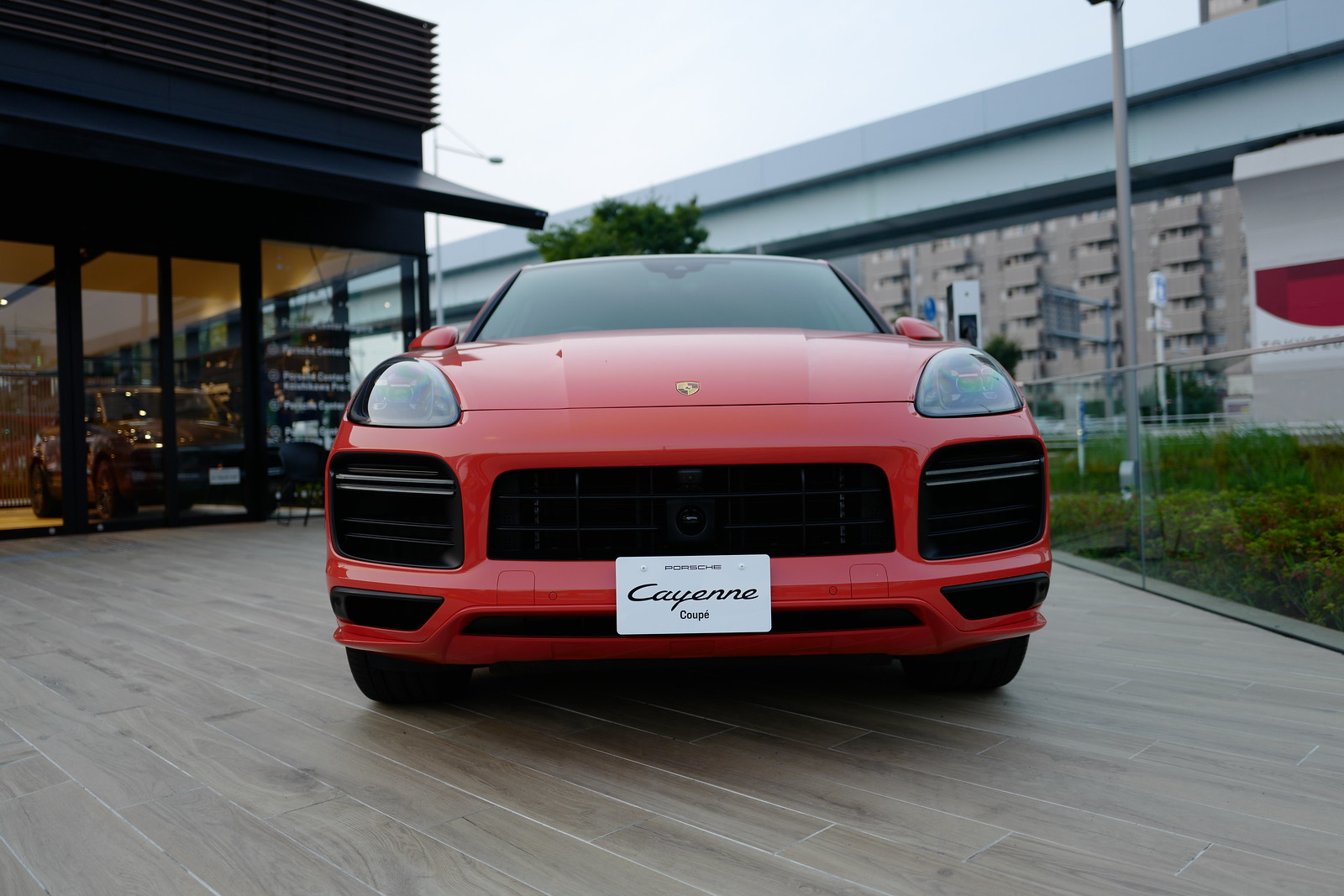This photograph captures a bright red Porsche Cayenne Coupe prominently positioned on a wooden deck outside a Porsche dealership. The car, facing the camera, displays a white license plate with "Porsche Cayenne Coupe" written in bold black letters. The iconic gold Porsche logo gleams on its hood. Behind the car, the dealership's modern exterior features black roofing and large glass windows that give a glimpse of another luxury car, appearing darker in color. To the left, the showroom's spacious, glass-paneled walls offer a clear view inside, while to the right, a patch of green grass adds a touch of nature to the setting. Beyond the dealership, there's visible activity with a nearby freeway bridge and a multi-tenant housing project in beige, accentuated by balconies and possibly a train track running between the two structures. The scene also includes distant warehouse buildings with trucks and loading docks, contributing to the bustling backdrop.